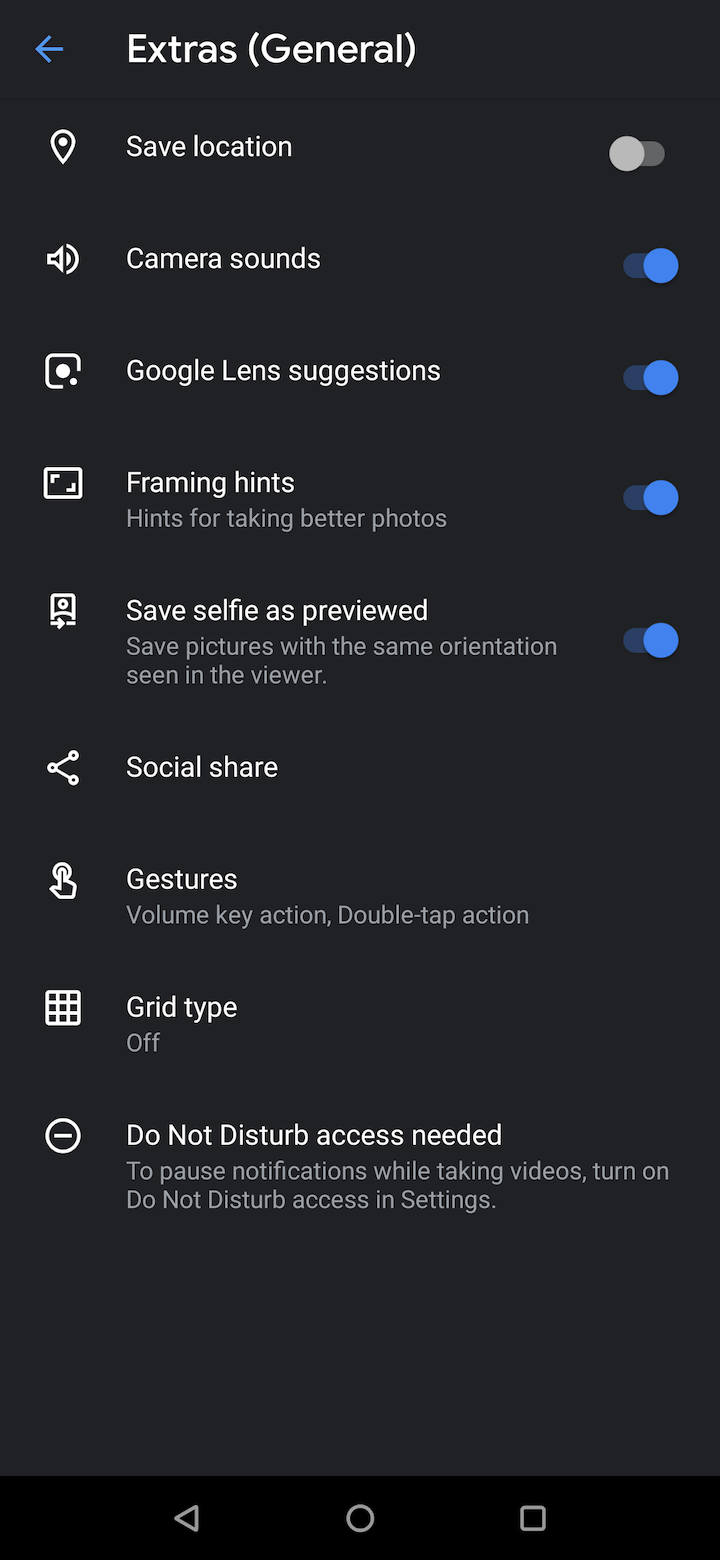This image is a screenshot capturing the "Extras" section within the "General" settings of a cell phone. The title "Extras" is prominently displayed on the upper left-hand side in a slightly left-justified format, accompanied by a blue back arrow to its left. 

Beneath the title, a series of menu options presents various toggle settings. The first option, "Save Location," is toggled off. The next option, "Camera Sounds," is toggled on. Following that is "Google Lens Suggestions," which is also toggled on. Below that, "Framing Hints," which includes the description "Hints for taking better photos," is toggled on. Finally, at the bottom, "Save Selfies as Previewed," with the additional note "Save pictures with the same orientation seen in the viewer," is also toggled on.

Each toggle provides specific functionality, enhancing the user experience based on personal preferences for saving photos, capturing sounds, and generating suggestions for better image framing.